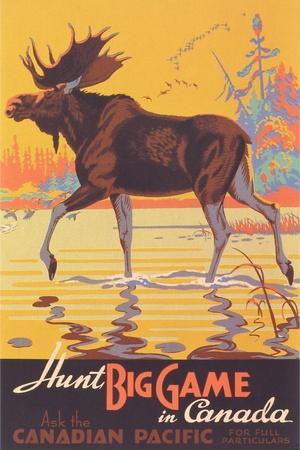The vertically aligned rectangular image resembles a vintage tourism poster for Canada, possibly serving as a book cover or promotional material. Dominating the center of the image is a cartoon-styled large brown moose with tan legs and prominent antlers, standing in shallow water, giving the impression of a subtle smile with its closed mouth and expressive eyes. The water below the moose has rippling pale yellow waves, interspersed with darker yellow zigzag lines, and occasionally some stones, hinting at motion.

Above the moose, the sky is depicted in a warm orange hue, suggesting a sunset, and is populated with birds in flight and a mix of orange, blue, and green trees. These elements create a serene yet adventurous atmosphere.

At the bottom of the poster, a bold black rectangular band houses the text. The first line reads "HUNT BIG GAME" with "HUNT" in a white script font and "BIG GAME" in orange uppercase printed font. The next line to the right says "IN CANADA" in the white script font. Below this, "ASK THE" appears in a thin orange font, and the final line "CANADIAN PACIFIC for full particulars" is in orange uppercase, with "CANADIAN PACIFIC" larger than the rest of the text.

Overall, the poster invites viewers to hunt big game in the picturesque landscapes of Canada, with specific details provided by the Canadian Pacific.